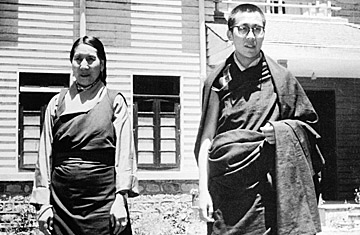This rectangular photo captures an outdoor scene featuring two people against the backdrop of a two-story wooden structure with a white awning providing shelter for a doorway. The structure, with its wood siding and two rectangular windows on the bottom floor, exudes a rustic charm. On the left side of the image stands a woman who appears to be of Asian descent. She is wearing a long-sleeved shirt and a dark-colored apron, giving her a professional yet approachable appearance. Next to her, on the right, is a man also of Asian descent. He has short hair and wears glasses, dressed in an attire reminiscent of a monk's traditional clothing. The man is gazing towards the right, adding a contemplative mood to the composition. The tranquil setting and the individuals’ attire suggest a serene, possibly spiritual context to the scene.